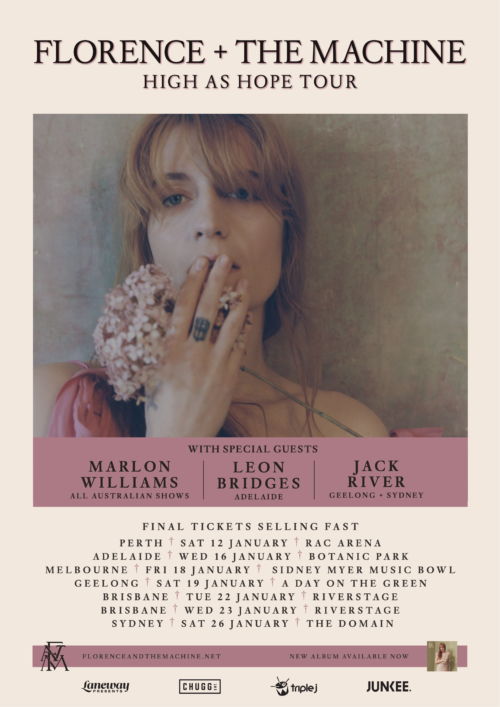This detailed promotional poster for the "Florence + The Machine - High As Hope Tour" is set on a light peach-colored background. At the center is a vibrant color close-up of a young woman with reddish-orange hair holding pink flowers in her right hand, wearing a low-cut dress and a tattoo on her middle finger. The poster prominently features the band's name and tour title at the top. Below the image, special guests are listed including Marlon Williams for all Australian shows, Leon Bridges for Adelaide, and Jack River for Geelong and Sydney. The tour dates and venues are: Perth at Rack Arena on Saturday, 12 January; Adelaide at Botanic Park on Wednesday, 16 January; Melbourne at Sydney Meyer Music Bowl on Friday, 18 January; Geelong at A Day on the Green on Saturday, 19 January; Brisbane at River Stage on Tuesday, 22 January, and Wednesday, 23 January; and Sydney at The Domain on Saturday, 26 January. It emphasizes that final tickets are selling fast.